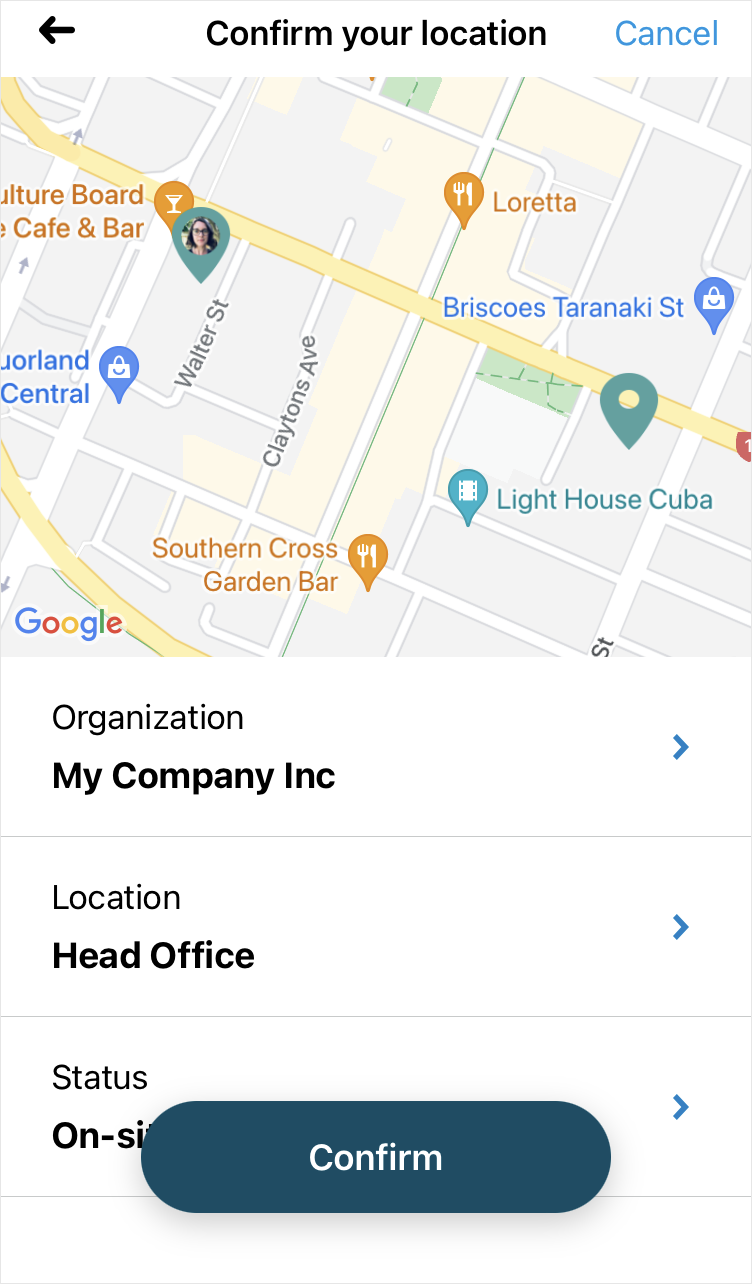This image features a user interface centered around a map to confirm a location. On the left side of the screen, an arrow pointing upwards is followed by a left-pointing arrow and the text "Confirm your location" in black. The right side displays the word "Cancel" in blue. The map itself dominates the center, with various colors including green, blue, orange, yellow, gray, tan, and teal, possibly indicating different regions or landmarks. 

Beneath the map, a section labeled "Organization: My Company" includes a right-pointing blue arrow and a gray line indicating "Location: Head Office," complemented by another blue arrow on the right side. Below this, partly obscured by a large teal "Confirm" button with white text, there's an indication of the status, which suggests "on site" but is partially covered. Various colored pins or markers are visible on the map, implying points of interest or specific locations, including a teal pin which might be significant. Another teal marker features an image of a woman with white skin, dark hair, and dark glasses. Hints of other pins or markers in red are also present, though their specific relevance isn't clear. The overall scheme incorporates white, black, and multiple shades of blue, teal, and gray, creating a vibrant yet structured interface.